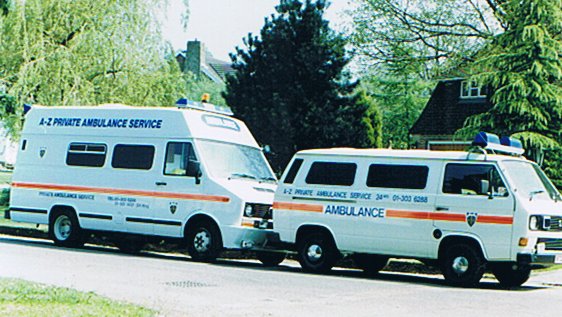In this vivid photograph taken on a sunny day, two white ambulances are prominently featured, positioned closely beside each other, possibly waiting at a red light. The larger ambulance in the background bears the label "A2 Private Ambulance Services" in blue letters at the top and features an orange stripe running along its side, complemented by black tires. This vehicle, with its higher front, resembles a large delivery van and hints at a spacious, more traditional ambulance design. The smaller, van-like front ambulance, also white, displays an orange stripe interrupted by the word "Ambulance" in blue letters, along with additional text above, likely including a phone number. Both ambulances have visible windows, blue emergency lights, and silver rims on black tires. Surrounding the ambulances are various green trees: a tall, light green willow in the top left corner, a darker evergreen in the center, and another dark tree on the right. In the background, behind the trees, are two houses, one featuring a dark brown roof and white-framed windows. The scene is completed by light green grass and yellow patches at the bottom left and stretches of light macadam road beneath the ambulances.